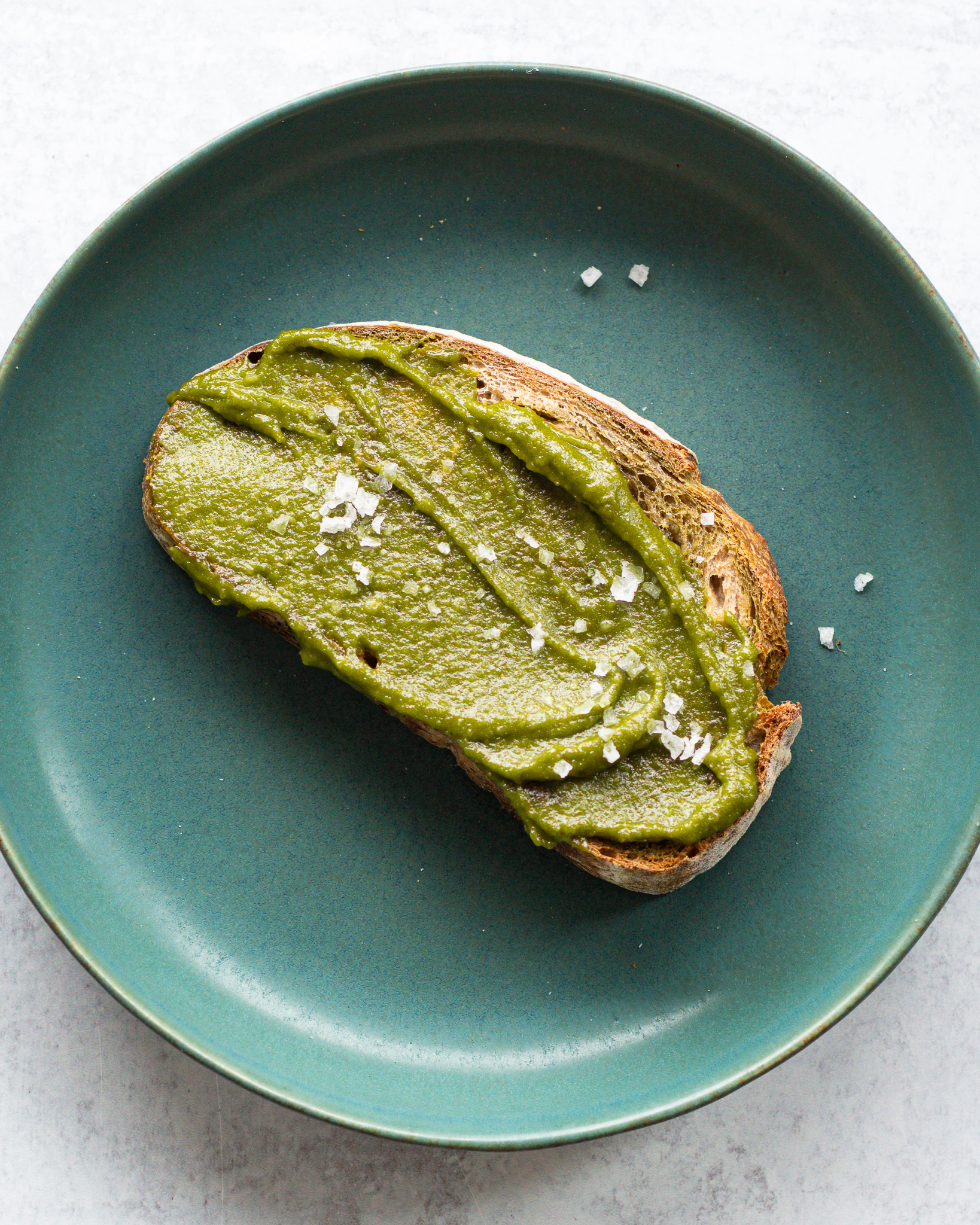The image showcases a round, circular, green plate placed on a subtly grained white surface. At the center of the plate lies a slice of toasted Italian or possibly sourdough bread, distinguished by its brown crust and scattered white flour. The bread is generously topped with a light green avocado spread, forming a smooth layer. Sprinkled atop the avocado spread are fine pieces of a white fruit, resembling coconut shavings or possibly sea salt. Additionally, four small chunks of this white fruit are delicately placed to the right of the toast, adding a finishing touch to the presentation. The plate's vibrant green hue contrasts beautifully with the white background, giving a clean and appealing aesthetic to the overall composition.